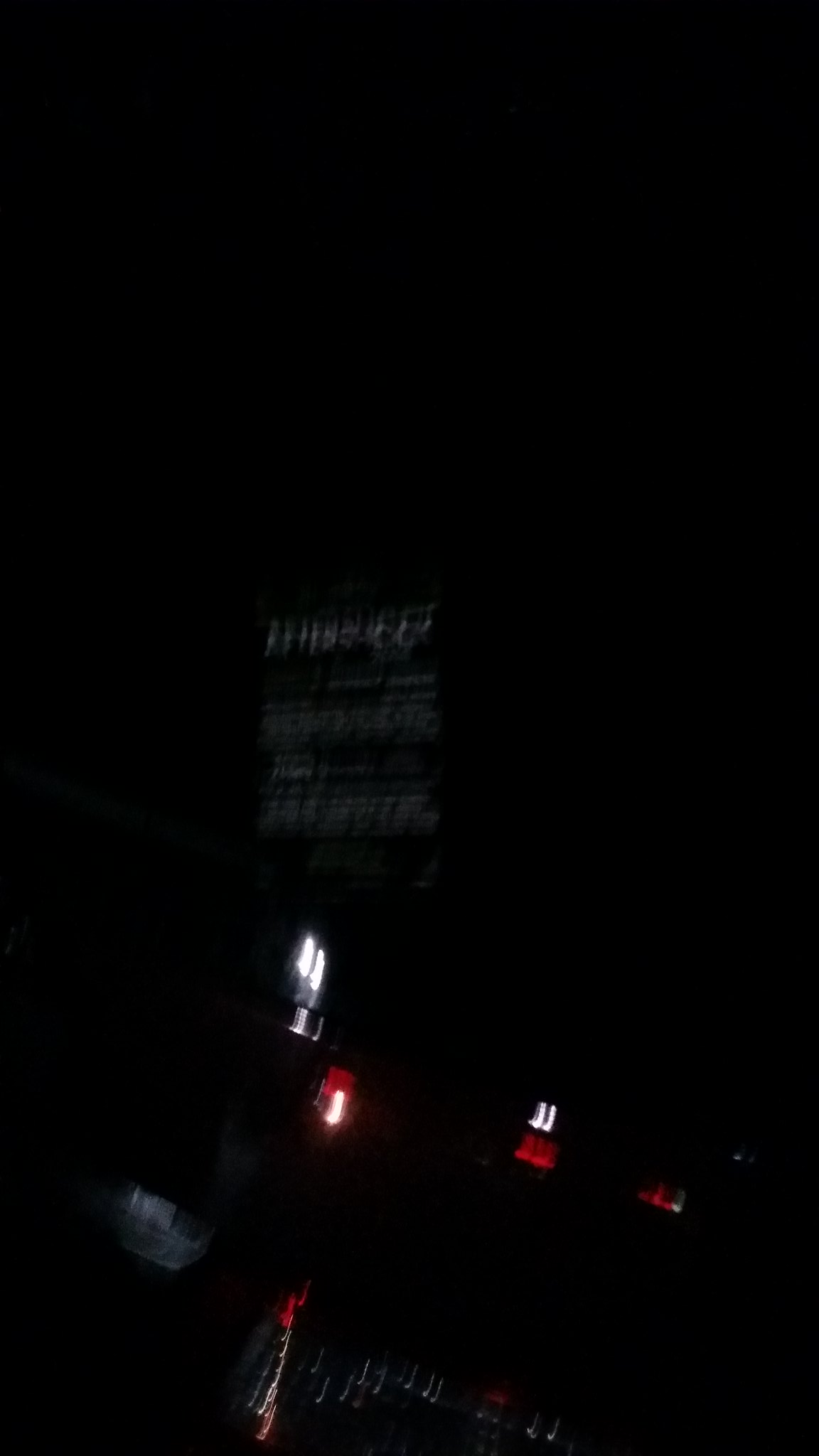This is an exceptionally dark and blurry color photograph, presenting an enigmatic and obscure scene. The central focus appears to be a structure that might be a billboard or a sign, casting an indistinguishable presence amidst the darkness. Below this central feature, there is an array of blurred white and red lights, hinting at the possibility of vehicles in motion or illuminated signage. The blurring effect at the bottom of the image particularly suggests dynamic movement within the frame. A prominent white blur occupies the left corner, further adding to the photograph's abstract nature. The overall composition is much taller than it is wide, contributing to a vertical emphasis. Due to the severe blurriness and lack of clarity, no specific objects or inscriptions can be clearly identified, making the image's content and context largely ambiguous.